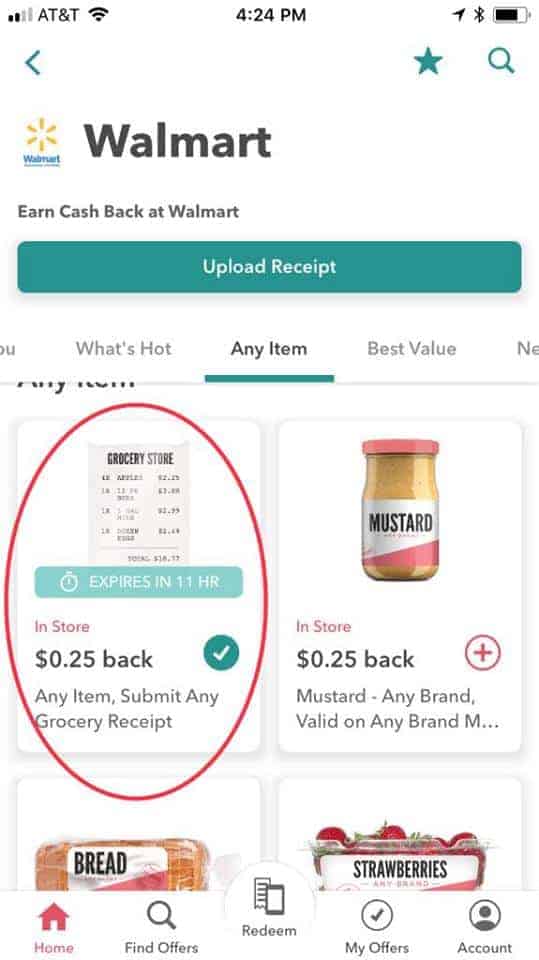This screenshot from the Walmart app provides a comprehensive display of its user interface at a glance. 

At the top left corner of the screen, the status bar shows the AT&T network icon, Wi-Fi signal strength, the time (4:24 p.m.), active Bluetooth connection, and battery status. Directly beneath the status bar, from left to right, there are navigational icons: a left arrow for returning to the previous screen, a star icon, and a magnifying glass for search functions.

Centered below these icons, the Walmart logo and the word "Walmart" are prominently displayed. Directly beneath the logo, there is a banner that reads "Earn cash back at Walmart" accompanied by a button labeled "Upload receipt."

Under the banner, three menu items are listed horizontally: "What's Hot," "Any Items" (which is currently selected), and a partially visible item starting with "Best Value," followed by a cutoff word that begins with "N."

The main content area of the screenshot showcases a collage of four items and their details. The top left corner displays a grocery store icon with captions that read "Expires in 11 hours," "In-store 25¢ back," "Any items," and "Submit any groceries receipt," all encircled by a red oval. To the right, an image of a mustard jar with a red lid offers "In-store 25¢ back, mustard, any brand" and mentions its validity on any brand. Below the mustard, the top of a bread package is visible with the word "Bread" written on it. The bottom right corner shows a package of strawberries labeled "Strawberries."

Finally, five menu icons are aligned at the bottom of the screen: "Home," "Find Offers," "Redeem," "My Offers," and "Account," providing navigation to different sections of the app.